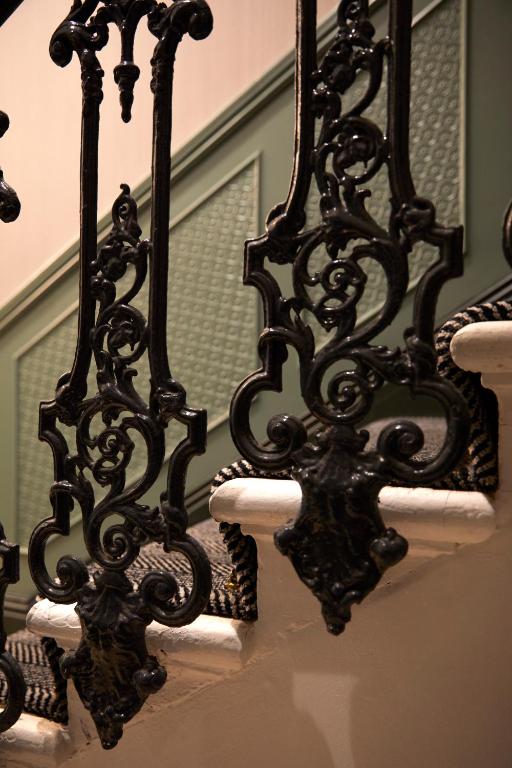The image depicts a close-up view of a staircase. The staircase is primarily white, likely painted, with a runner of black and white braided or striped carpeting adorning the treads. The railing is decorative and wrought iron, painted black, featuring intricate welded designs including circles and squares, and is fastened to the sides of the steps, which appear to narrow as they ascend. The banister itself is also black. The backdrop consists of a wall painted in a light army or grayish-green color, segmented by wooden frames that create square patterns, adding texture to the scene. The staircase starts at both lower corners of the image and rises toward the center, with the wall extending diagonally behind it. The setting suggests an interior within a building.